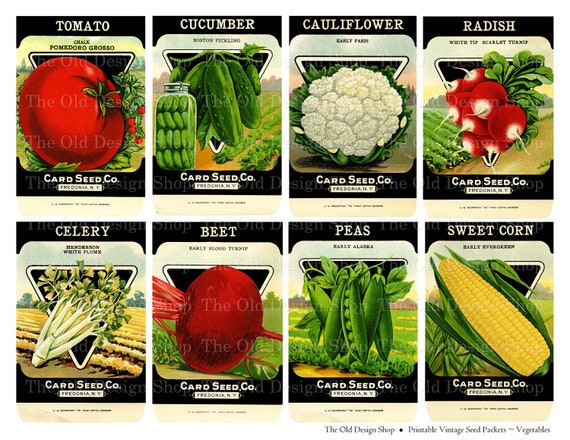This vibrant advertisement for Card Seed Company features a collection of eight seed packets arranged in two rows of four. Each packet showcases a vivid illustration of the mature vegetable it contains, creating an enticing visual display. The top row includes a bright red tomato labeled "Pomodoro Grosso," green pickling cucumbers, a large yellow cauliflower head, and scarlet turnips alongside white-tip radishes. The bottom row displays ivory-colored celery, a bright red beet, vivid green pea pods, and a yellow ear of sweet corn. The label "Card Seed Company, Somewhere, New York" appears on each packet, making this collection an ideal starter pack for a summer vegetable garden, perfect for spring planting.